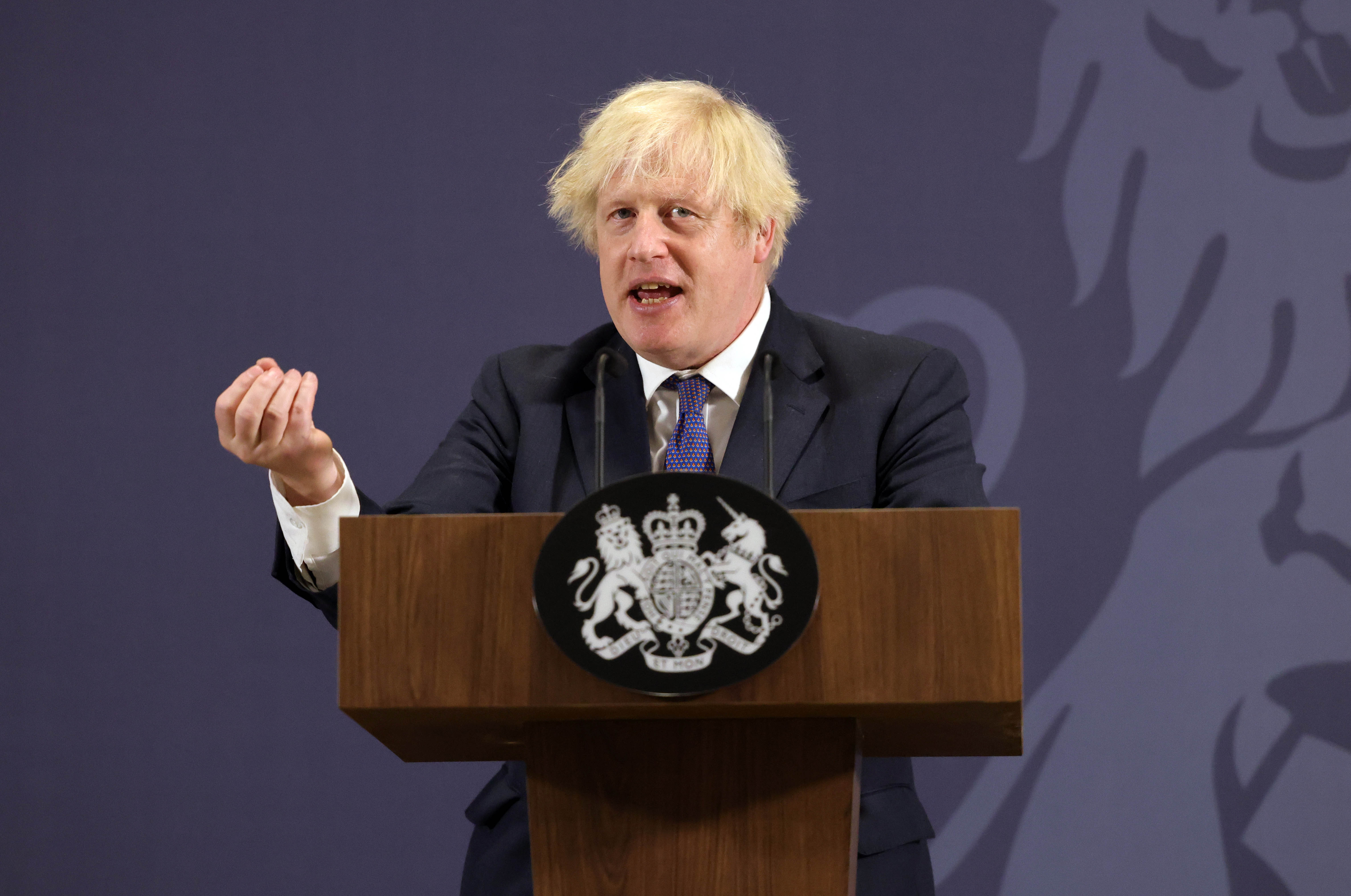This image captures Boris Johnson, the former Mayor of London and Prime Minister of the UK, standing behind a wooden lectern adorned with a black oval plaque bearing a crest that includes a lion, a unicorn, and a crown. He is framed against a background featuring two shades of blue, with a subtle design that mirrors elements of the emblem on the lectern, including a discernible lion's mane and tail. Johnson, with his distinctive shaggy blonde hair and characteristic bad haircut, is dressed in a dark suit, white shirt, and a tie that's been described as both blue-patterned and purple. His mouth is open as he appears to be speaking, and his right hand is raised, fingers and thumb together, gesturing to emphasize his point.